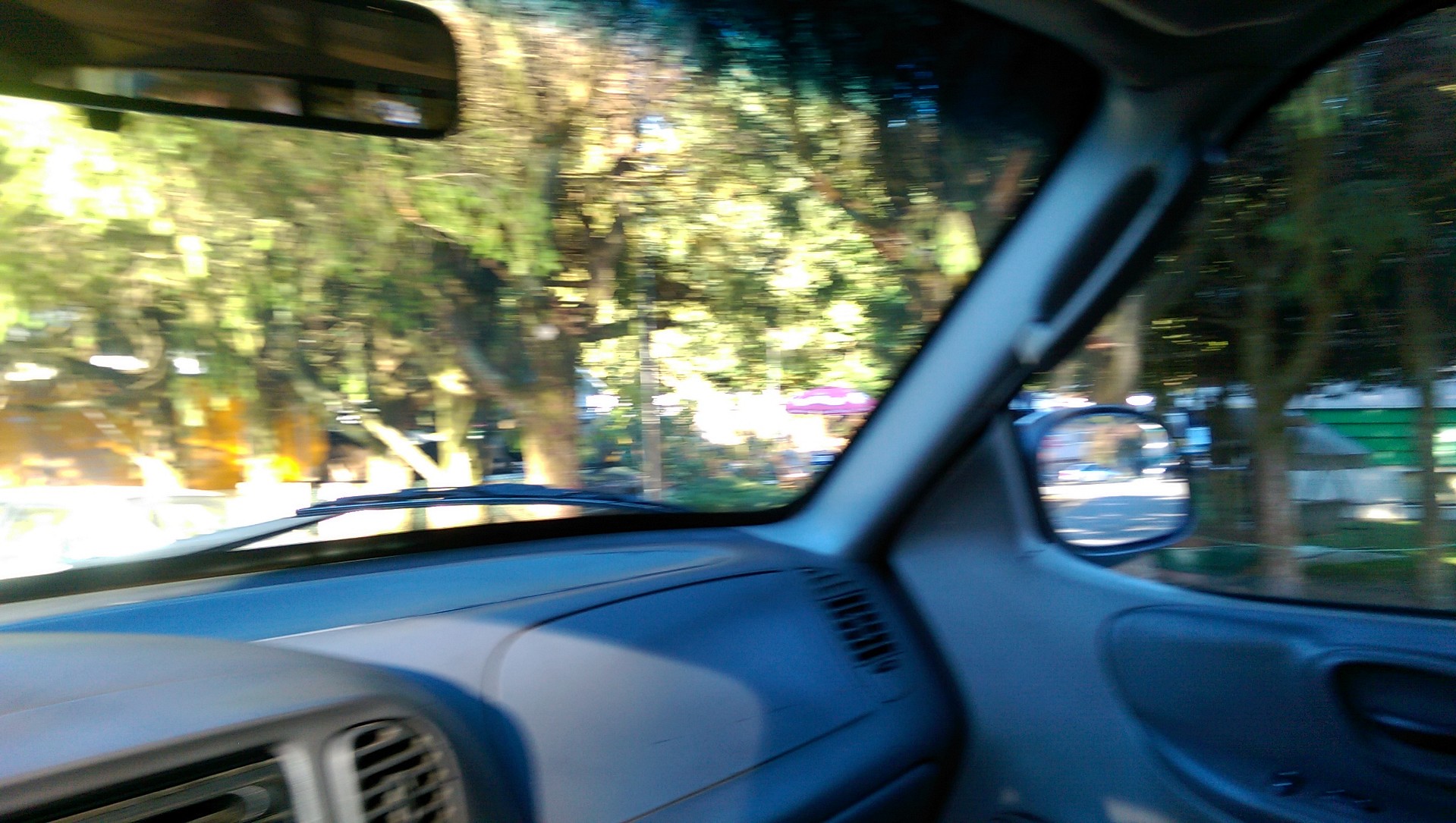A blurry image captured in landscape aspect ratio, potentially a still frame from a video, showing the interior of a moving car. The photo is taken from the perspective of the driver and is aimed towards the front right corner of the vehicle, encompassing the passenger seat, dashboard, and the view through the window. The car’s interior is adorned in cool gray tones, featuring air vents, glove compartments, and various dashboard elements. Outside the window, the background reveals a blur of green trees, enhanced by the motion blur, indicating the car's movement.